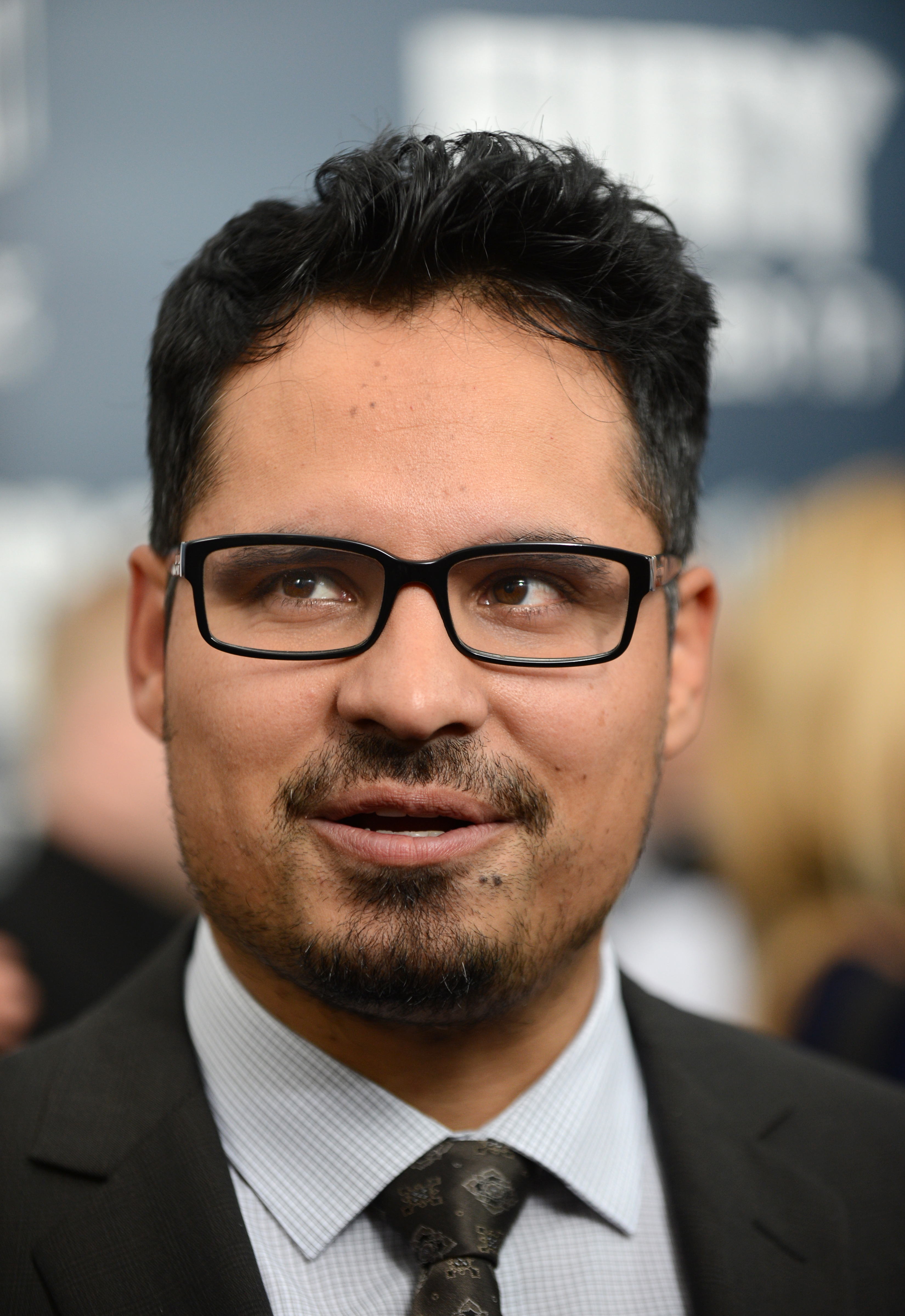In this close-up photograph, a man, who appears to be actor Michael Peña, is the focal point. He is dressed in a dapper black tuxedo, accented with a collared, white dress shirt featuring a subtle blue stripe pattern and checker or square textures. Over this shirt, he dons a light gray tie with a diamond-like print, though primarily gray in appearance. His facial features include thick, black-rimmed, square glasses, brown eyes, and short black hair that is gelled and brushed back, giving a slight wavy texture on top. He sports a very thin mustache and a sparse beard, prominently around his lips and chin. The backdrop is completely blurred but hints at a white logo or text along with indistinct figures, suggesting the presence of a crowd. In this image, he looks slightly to the left with a serious expression, his mouth slightly open, adding an element of candidness. This well-framed portrait captures both his stylish attire and his charismatic presence amidst an indistinct background scene.